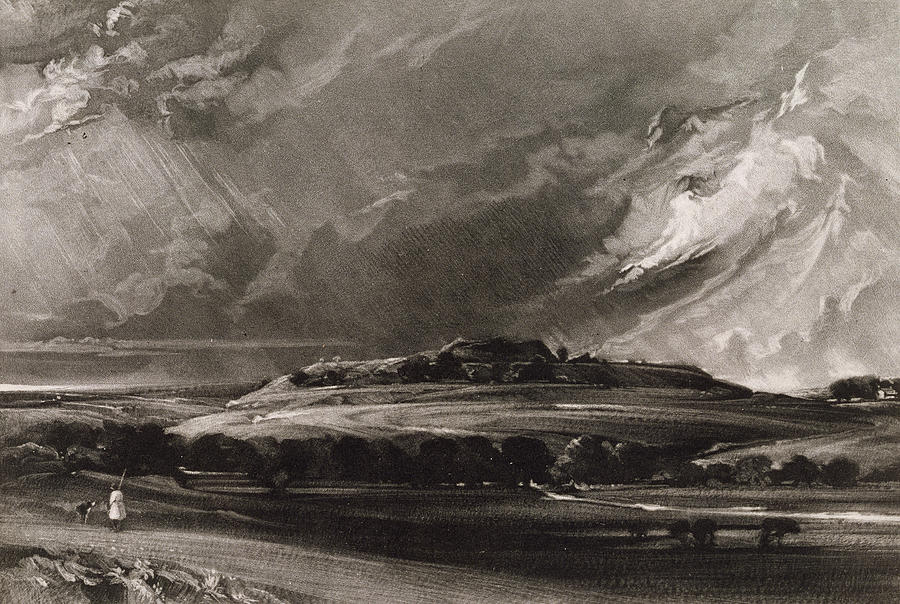This grayscale painting depicts a desolate plateau valley under a violent storm with dramatic cloud formations that dominate the sky. The clouds are dark and swirling, appearing almost like waves crashing over the landscape and streaks of what may be either torrential rain or rays of light pierce through them, creating a striking contrast. In the lower left-hand corner, a shepherd kneels beside his dog, both of them facing the storm yet making no attempt to seek shelter despite a nearby house and barn on the far right side of the image. The barren yet grassy fields are dotted with multiple trees, and central to this scene is a distinct flat-topped hill rising amidst the valley, emphasizing the foreboding nature of the stormy backdrop. The entire scene evokes a powerful sense of nature’s fury and human resilience.